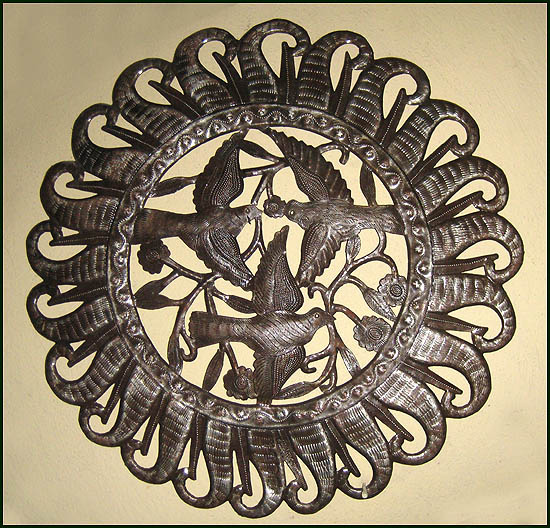The image showcases an intricate metal artwork, primarily in a dark bronze, brown color with a rich texture. The artwork features three small birds centrally positioned, two at the top facing each other with outstretched wings almost touching, and a third bird at the bottom appearing to fly away with one wing up, brushing against the lower bird's wings. Surrounding the birds are delicate vines adorned with roses, interspersed with leaves and branches. Encasing the central design is a circular ring with a wavy line and dot pattern, extending into a radiant, sun-like structure with alternating points and spirals. All elements appear meticulously crafted, contributing to the overall elaborate aesthetic. The piece is set against a solid tan background, emphasizing its detailed craftsmanship and ornate design.